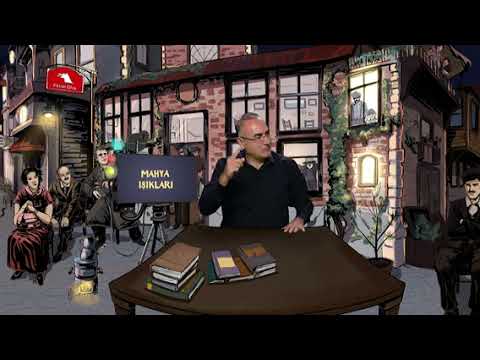In the image, a bald man with light skin and glasses is seated at a cartoonishly drawn brown wooden table, covered with similarly styled books, positioned towards the left hand top corner. He is centrally framed, wearing a black button-up shirt. Behind him, the background appears digitally rendered and resembles an old red brick city with glowing yellow windows and storefronts, and a sign that reads "Mahia Iskallari." Surrounding the main figure, there's an assortment of people: on the left, a woman in a long burgundy dress and two men, while on the right, another man dressed in black appears to be taking a photo with an antique camera. The entire scene, bordered in black at the top and bottom, evokes a blended reality of cartoony digital art with an old-time aesthetic flourish.